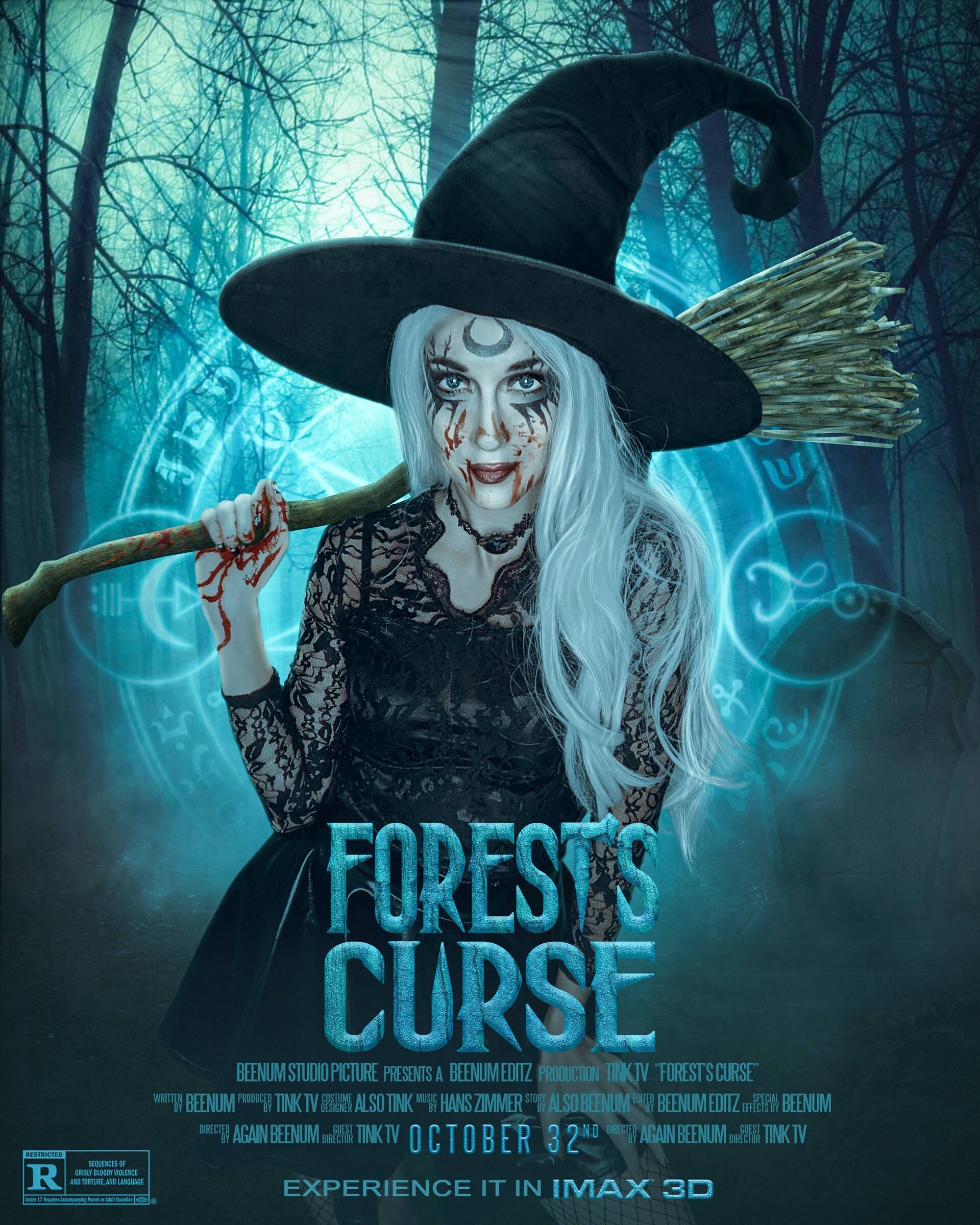This is a vertically aligned rectangular image, resembling a movie poster. The focal point is a witch with long white hair cascading over her left shoulder, adorned in a large black witch hat that curls at the ends. Her attire is a black lacy dress. She holds a blood-streaked broom over her right shoulder, the straw end angled to the right and the handle to the left, with blood dripping down her hand. Her face is marked with black symbols and she wears red lipstick, with additional blood spatters visible on her face. In the background is a dark, mystic forest with a bluish-teal hue, barren tree trunks closely packed together, and hints of light filtering through. Centered at the bottom is the movie title, "Forest Curse," followed by production credits and the intriguing date of October 32nd. The poster also advertises the experience in IMAX 3D and has a "Rated R" indication in a small rectangular box at the lower left corner.